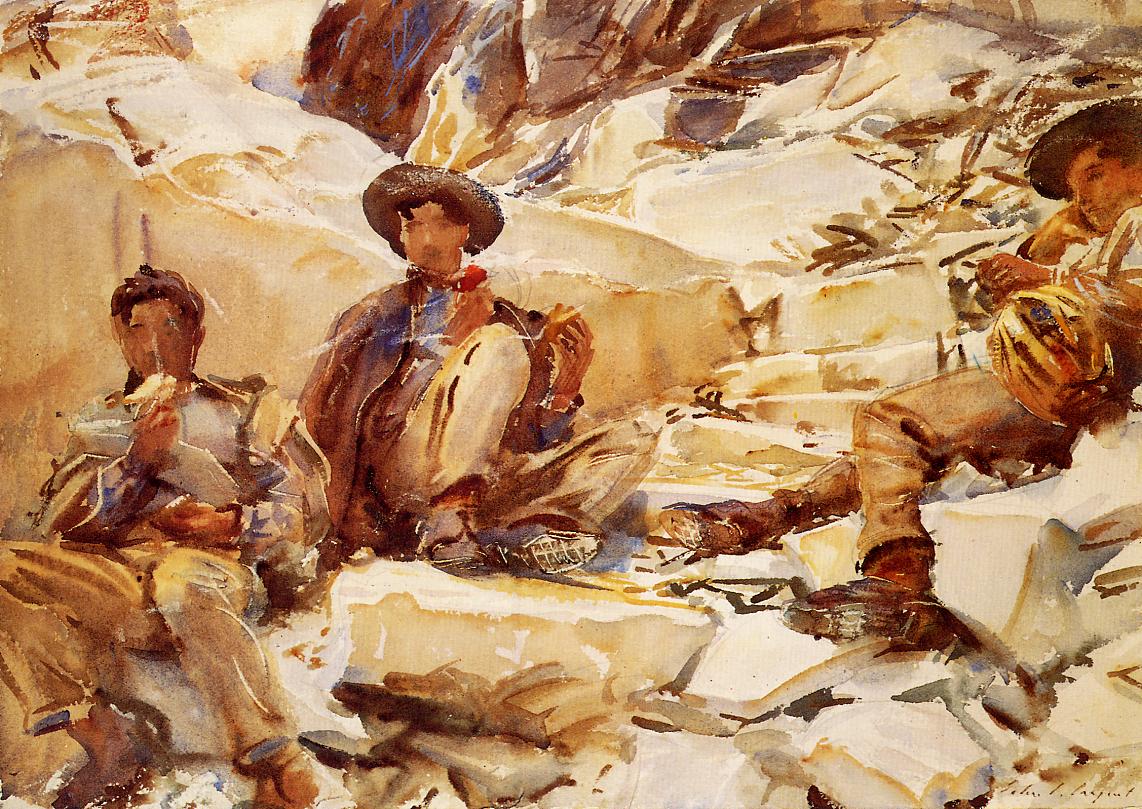The painting portrays three men dressed in attire reminiscent of workmen or cowboys from over 50 years ago, positioned on a rocky, hilly landscape. Executed in an impressionistic style using a minimal color palette of browns and tans, the details are vague but discernible. The man on the left, whose face is blurred, seems to be eating something white with his arm bent towards his face. The central figure, knees drawn to his chest, holds an apple and wears a hat. The man on the right, also hat-clad, lounges leisurely on a slope, examining something in his left hand. The figures are set against a backdrop of sandy, rocky terrain with visible steps or stones leading up the cliffside, contributing to the rough and simplistic feel of the piece. The overall composition captures a casual moment, possibly during a meal break, in a rugged environment.